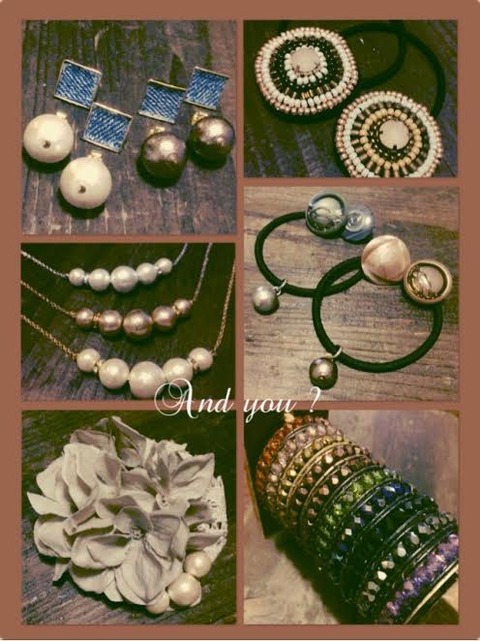The image features an array of various pieces of jewelry displayed in a 2x3 grid against a solid dark pink background, which acts as a border between the images. Each piece is placed on a dark brown wooden surface, showcasing the natural wood grain. In the upper left corner, two pairs of dangle earrings are featured: one pair with white beads and blue squares, the other with brown beads and blue squares. Directly below, three necklaces are displayed, each with five beads; one necklace has white beads, the second has brown beads, and the third has white beads again. In the bottom left corner, a floral jewelry piece, perhaps a pin, made of light pink petals with bead accents is presented.

The upper right corner holds a pair of hoop earrings adorned with light and dark brown circular beads. Below this, another set of hoop earrings features two large beads each, with one pair having gray beads and the other pair light pink beads. The bottom right corner showcases several colorful bracelets lined up next to each other in shades of purple, black, blue, green, brown, pink, and orange. Approximately two-thirds down the image, cursive white text reads, "and you?"